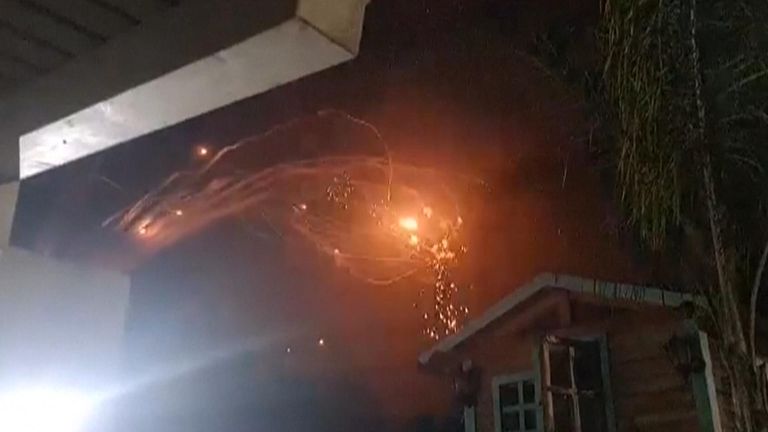The image features a night scene captured in landscape orientation, with a dilapidated, small wooden house or shed in the bottom right segment, which appears to be a light orange color with a white roof. The structure has a cross-paned window and door, indicating its rundown state. Above the house, to the left, a large tree extends its leafy branches over the roof. In the center of the image, there are mysterious sparks of light, likely indicating either a fire or fireworks, creating a dramatic effect with streaks of light and some visible smoke. The top left corner of the image features the under eaves of a building, adding to the outdoor ambiance. Off to the right, we can see green trees, possibly palm trees, that are not on fire, providing a stark contrast to the illuminated sparks in the middle. The overall scene is somewhat blurry, suggesting it was taken from a close vantage point, perhaps a porch, emphasizing the night-time setting and the potentially alarming central light display.